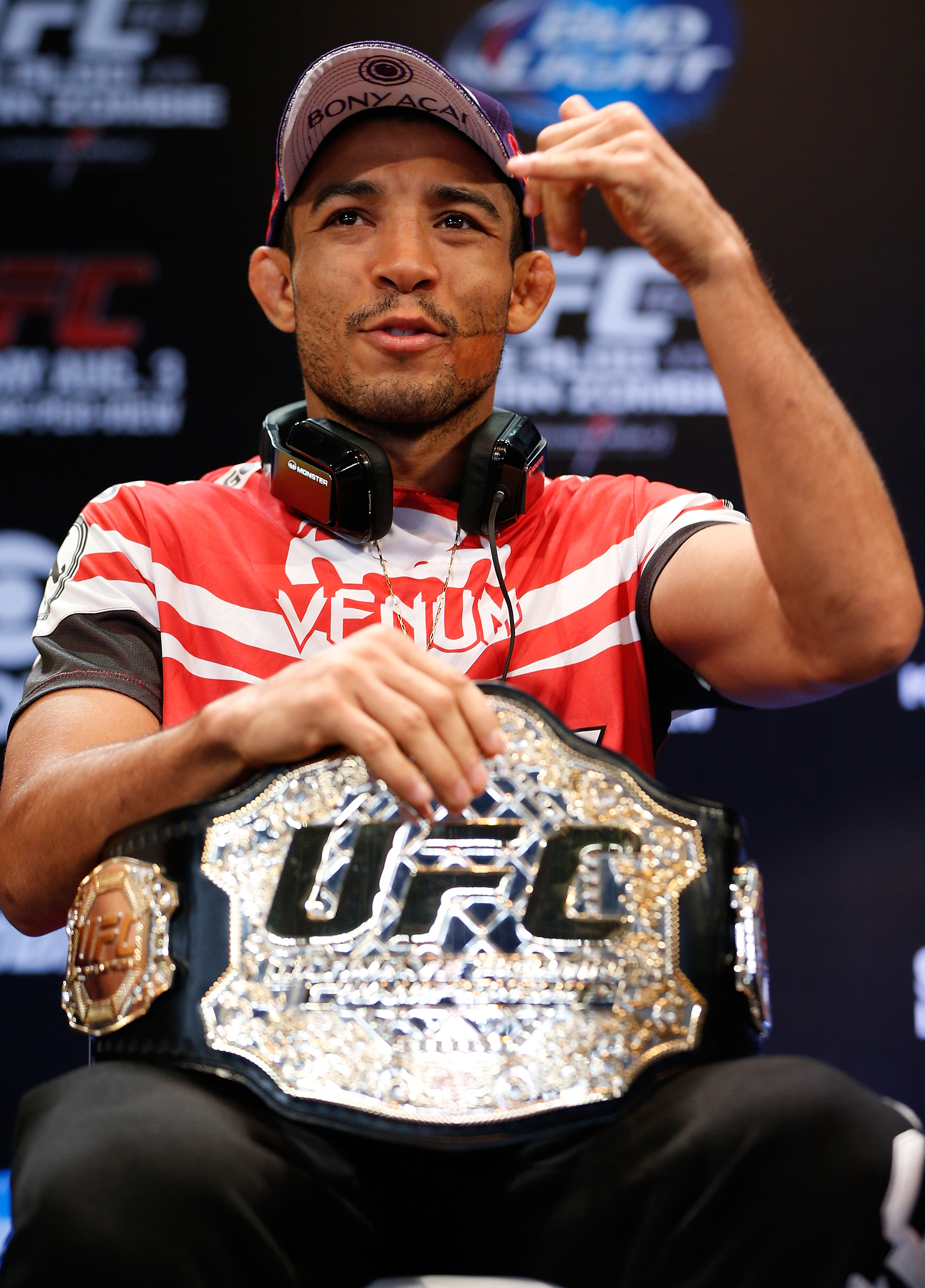In the photograph, a dark-complexioned man is seated, wearing black sweatpants and a red shirt adorned with white stripes through the center and black trim on the sleeves. The shirt features the word "Venom" near the neckline with an illustration of a snake's top half skull above it. He sports a blue baseball cap with a white underside on the bill that reads "BONYACAI," and over-the-ear headphones with a black wire rest around his neck. The bill of the cap partially obscures his dark hair, which is only slightly visible at the sides. 

In his lap, he holds a large black leather belt with a substantial, shiny gold buckle emblazoned with "UFC." He's gripping the belt with his right hand, while his left hand, bent at the elbow, is raised near his face as if he's gesturing while speaking. The man also has a bit of a mustache and beard, and his mouth is open, suggesting he is in the midst of talking. The photograph prominently captures his striking attire and detailed accessories.